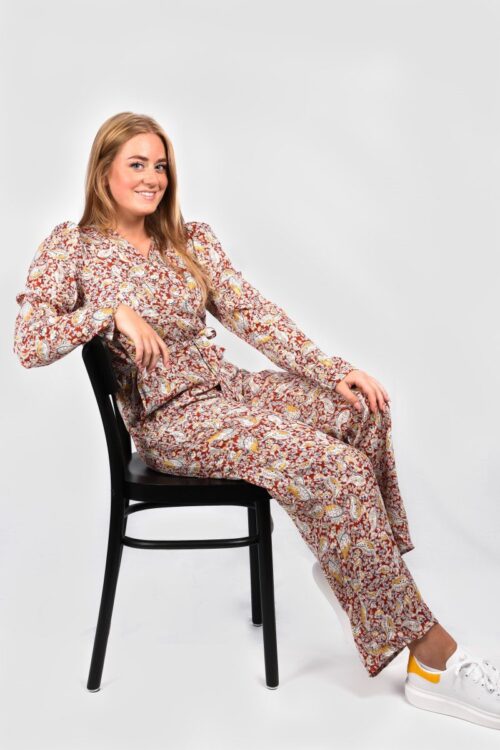The photograph depicts a woman seated on a black, four-legged chair with a circular band connecting the legs at the top, and small silver caps on the bottom of each leg. She is situated against a gray wall with a white floor beneath her, giving the impression of her sitting in an empty white void. The chair has a solid black seat cushion and backrest, and the woman, with shoulder-length dirty blonde to brown hair featuring a hint of bronze, is twisting slightly to her right while looking directly at the viewer with a big smile and open mouth revealing her white teeth.

She is wearing a vibrant, one-piece paisley jumpsuit adorned with an array of colors including white, red, blue, and brown, and zipped in the front. Her right arm is relaxed and resting on the top of the chair, just below her wrist, while her left hand clasps her left knee. The woman’s left leg is bent, and her right leg is more extended with part of her white tennis shoe—marked by white laces and a yellow band at the heel—visible, though the tip of her right toes is cropped out of the frame.